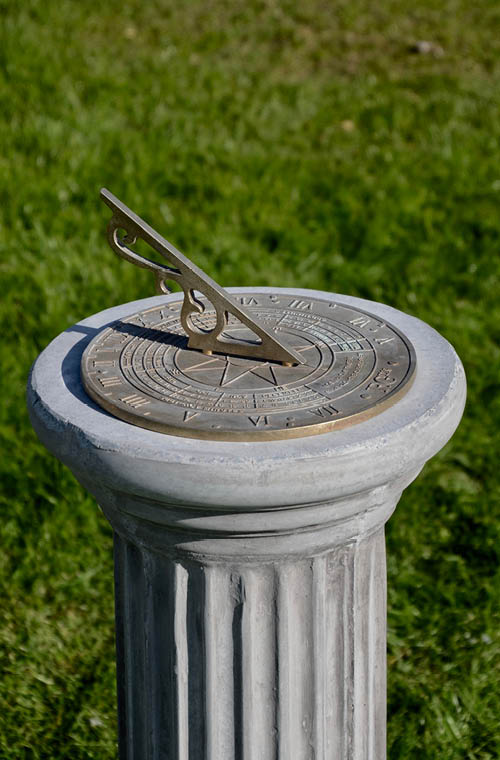A sundial sits atop a small, gray concrete column amidst vibrant, healthy turf grass on a sunny day. The sundial, crafted from oxidized brass that has developed green patches, features a sunburst at its center from which a pointed gnomon extends. The Roman numerals encircle the edge of the dial, which measures time by the shadow cast from the gnomon. The gnomon itself has a long, arrow-like design with intricate scrollwork at its base. This historical timekeeping instrument elegantly melds functionality with decorative artistry.